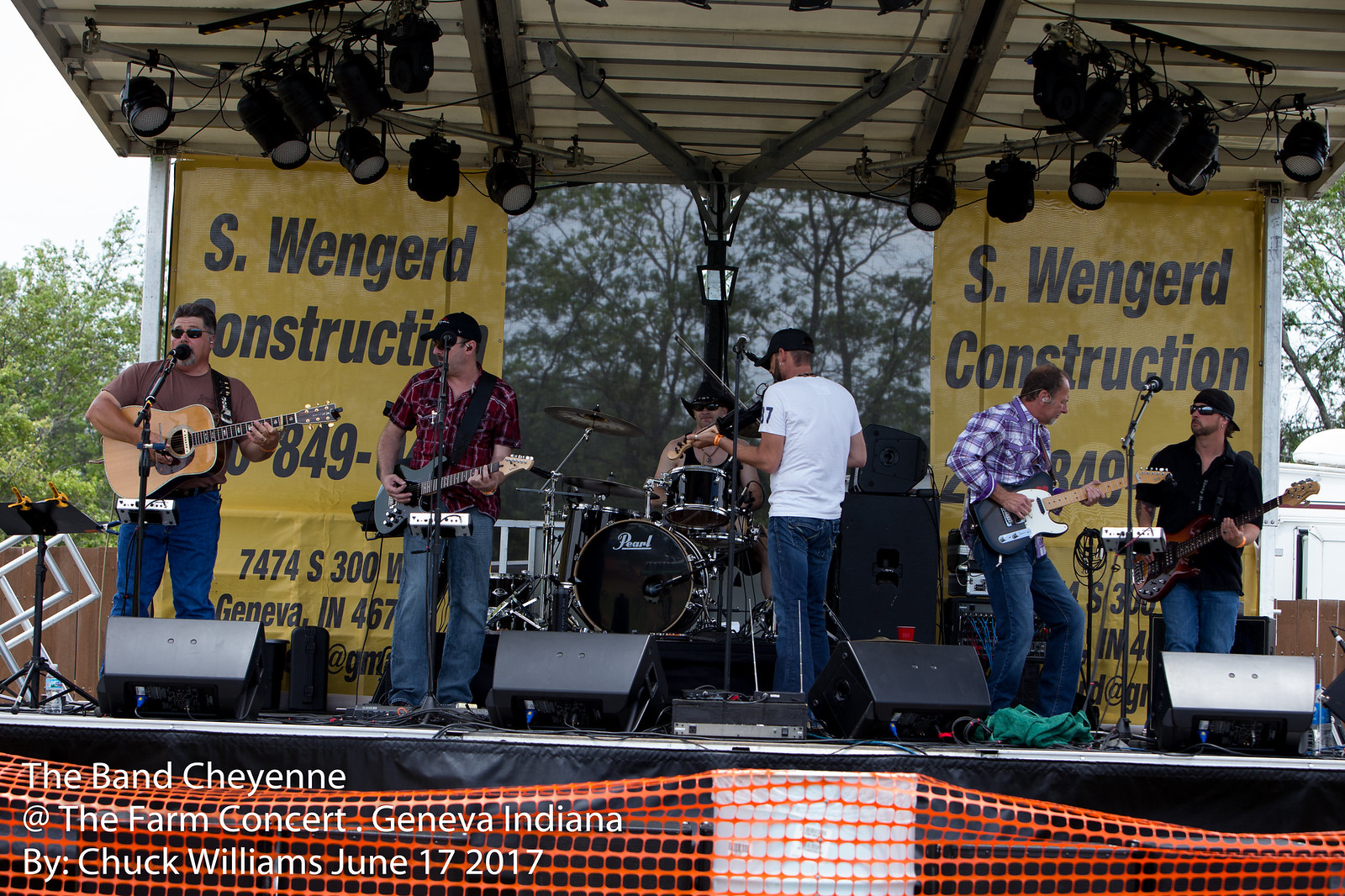This full-color photograph captures an outdoor summer concert featuring the band Cheyenne at the Farm Concert in Geneva, Indiana, on June 17th, 2017. The horizontally aligned rectangular image shows a stage with a canopy adorned with numerous spotlights. The background displays lush, leafy trees. Horizontally aligned, the stage is framed by yellow signs with black text from S. Weingard Construction, partially showing a phone number and address.

On stage, there are six musicians: the far-left guitarist, wearing jeans and a t-shirt, sings into a microphone. Next to him stands another guitarist in jeans and a plaid button-down shirt, looking at the first. Central to the stage, the drummer, in a black tank top and cowboy hat, is flanked by the lead singer, who has his back to the camera, wearing jeans, a white t-shirt, and a black baseball cap while facing the drummer. Toward the right, another guitarist in blue jeans and a plaid button-down handles his instrument, and the far-right musician, in jeans and a black button-down shirt with a backward black baseball cap and sunglasses, completes the lineup. Each musician has a microphone. At the bottom left of the image, white text reads, "The Band Cheyenne at the Farm Concert, Geneva, Indiana, by Chuck Williams, June 17, 2017."